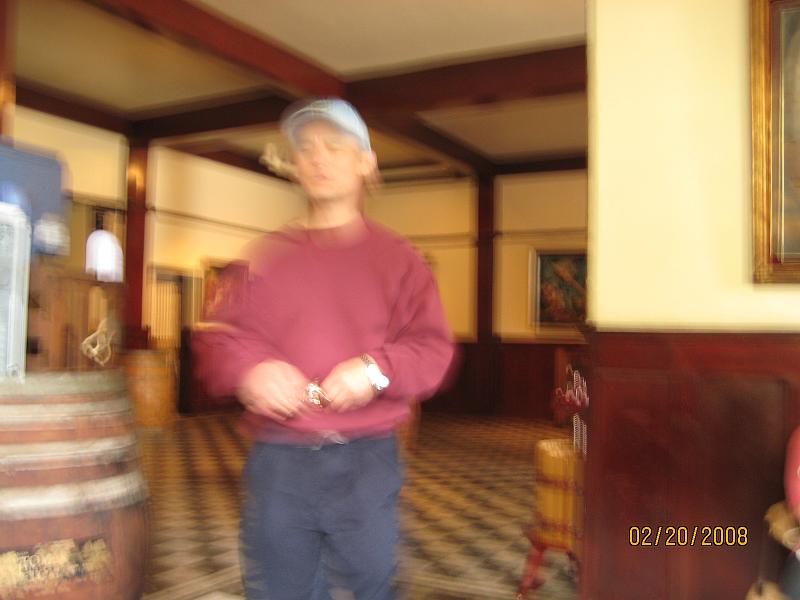A photograph dated February 25, 2008, features a room with distinct elements. In the bottom right corner, yellow text displays the date. The top right of the image shows a white wall adorned with a golden frame. The floor is covered in a black and white checkered pattern, contributing a classic feel to the space. Noticeable on the bottom of the image is a wooden area, juxtaposed against the rest of the scene. The background consists of various white walls and additional frames scattered around, particularly noted on the left side.

In the foreground on the left side, a barrel wrapped with white straps stands prominently, sporting a label facing the viewer. Above, wooden beams stretch across the top, interspersed with white squares that add to the design. Dominating the foreground is a person dressed in a red shirt and black pants, wearing a watch on their left wrist and a white baseball cap. The cap features closed highlights. The image bears a watermark at the top, possibly from a tool or website, reading "www.LRCgenerator.com."